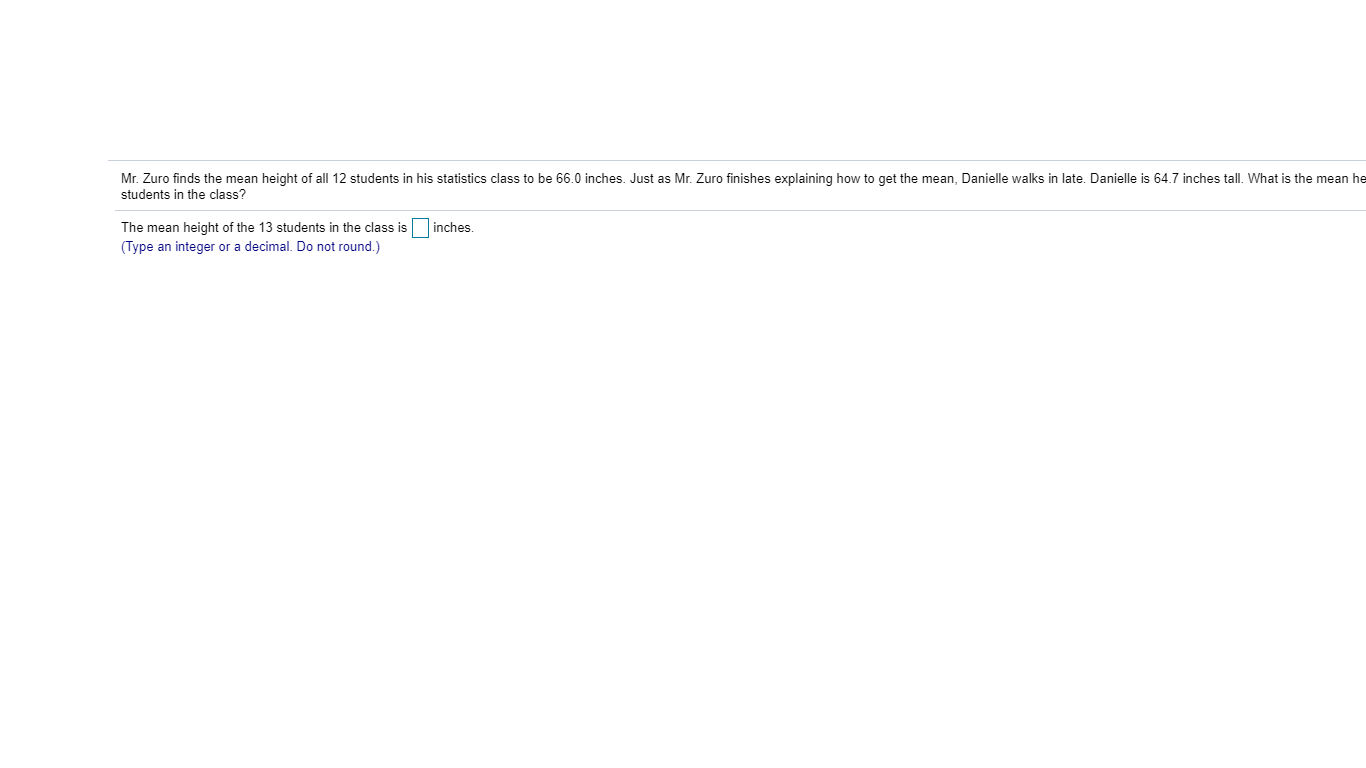The image is a narrow, horizontally oriented frame, partially cut off on the right side, displaying a question from an electronic test against a white background. The question is bordered by thin horizontal lines, either pale blue or light gray, both above and below it. The text reads:

"Mr. Zuro finds the mean height of all 12 students in his statistics class to be 66.0 inches. Just as Mr. Zuro finishes explaining how to get the mean, Danielle walks in late. Danielle is 64.7 inches tall. What is the mean he..."

The rest of the question text is cut off due to the frame's limitation. Beneath the bottom line, the text continues:

"The mean height of the 13 students in the class is _____ inches (type an integer or decimal. Do not round)."

An input box is provided for the answer next to the word "inches."